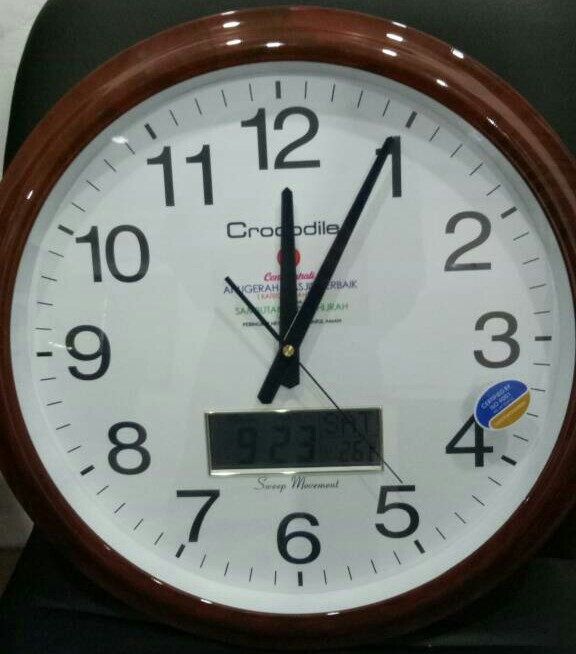This close-up photograph captures the face of an intricately designed clock set against a pitch-black background. Encircling the clock is a richly colored reddish-brown case, which beautifully contrasts with the pristine white circular face. Dominating the face are large, bold black numbers that clearly mark each hour. The time is precisely indicated with distinct black hands: the shorter, darker one for the hour, the longer, lighter one for the minutes, and a sleek black second hand. Subtle minute marks extend beyond the numbers, contributing to the clock's detailed design. Just below the center, straddling numbers five, six, and seven, lies a sophisticated black rectangle outlined in silver, offering an interesting highlight. Adding a splash of color, an oval label—blue on the top and brown on the bottom—finds its place between the numbers three and four, augmenting the clock's distinctive charm. The clock reads exactly 12:05, capturing a moment frozen in time.